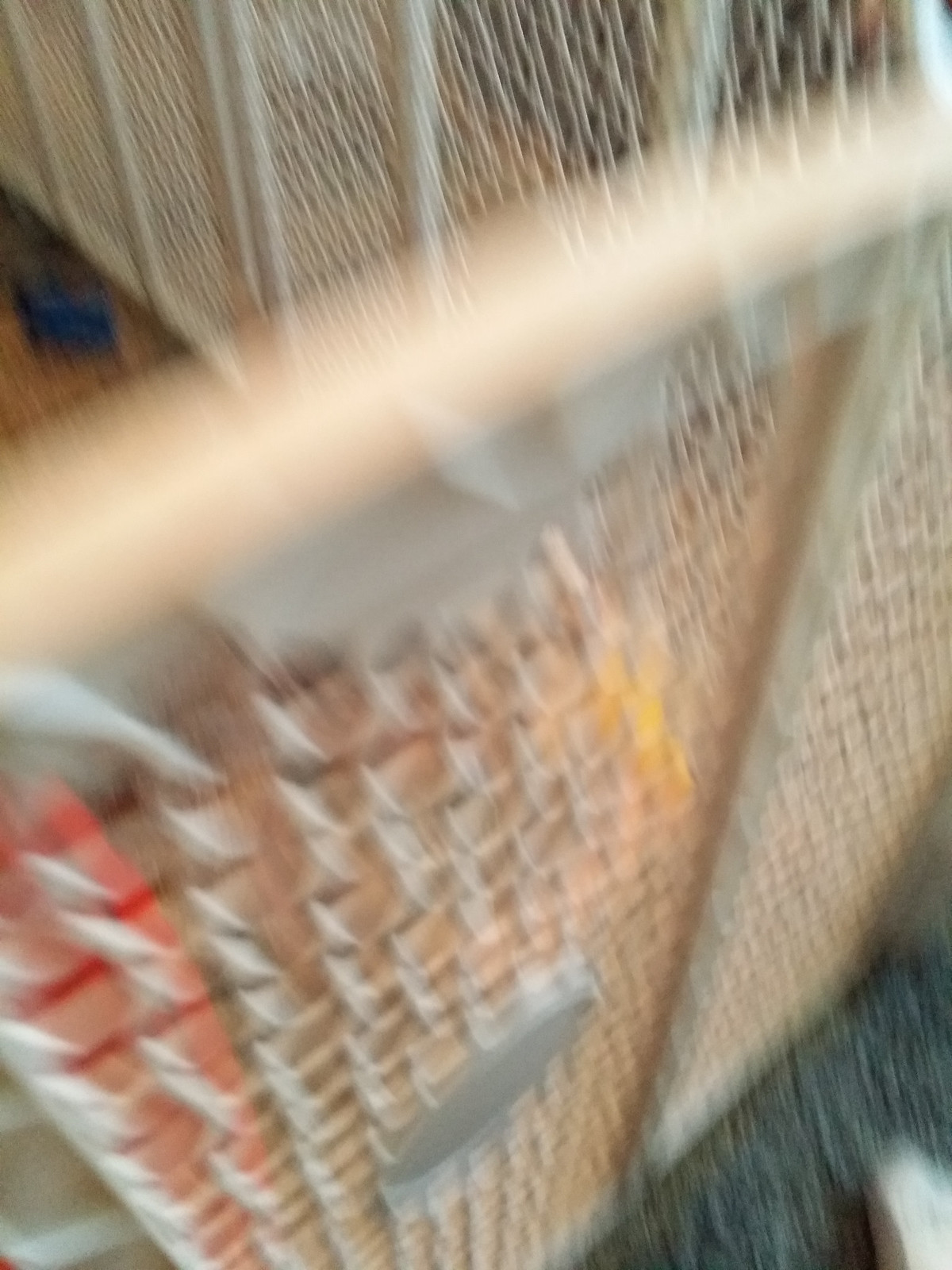The image showcases a blurry interior setting dominated by what appears to be a baby gate or a playpen. The gate, constructed from white plastic featuring brown wooden slats, occupies the foreground and background of the frame, creating a layered effect. A white railing runs along the top of the gate, adding to its structural detail. The lower right corner of the image reveals a patch of gray carpet, while the upper sections show brown carpeting, both indicating different flooring types within the home.

Interspersed throughout the scene are various colored objects, likely toys, hinting at the presence of a child. Specifically, a red object appears in the lower left corner, a yellow object is prominently placed in the middle, and a blue item is visible in the upper left corner. The overall blurriness of the picture makes it challenging to discern precise details, but the arrangement suggests a domestic environment organized for child safety and play.